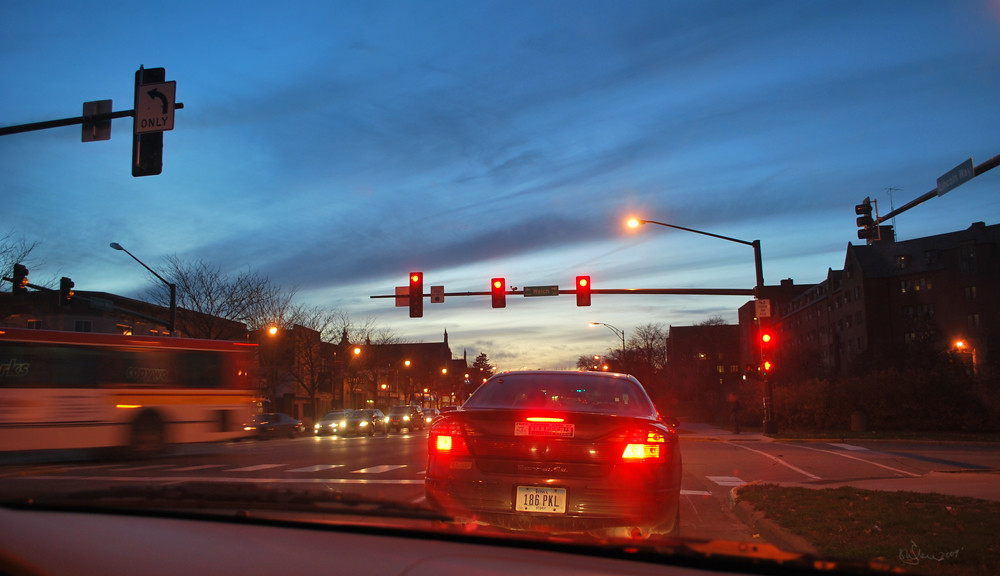The photograph captures a detailed scene from within a car stopped at a traffic light at night. The view is from the right side of the roadway, looking toward another vehicle directly ahead, displaying the license plate 186PKL. The car’s brake lights glow red, with a horizontal bar across the boot. 

Above the traffic, a horizontal bar supports three red traffic lights, and an additional red light is mounted on a vertical pole to the left of the stationary car. The opposite lanes are also filled with stopped cars illuminated by red lights and headlights, emphasizing the late dusk setting. A bus with a noticeable motion blur is making a right turn across the intersection.

The sky, transitioning from day to night, is a deep bluish hue with dark grey streaky clouds, suggesting an almost night-time but still slightly lit horizon. Streetlights are intermittently positioned along the left side of the image and one above the traffic lights to the right. Buildings, possibly hotels, restaurants, or shops, are faintly visible in the background, standing two or three stories high. This gives a sense of a vibrant yet halted moment in an urban setting.